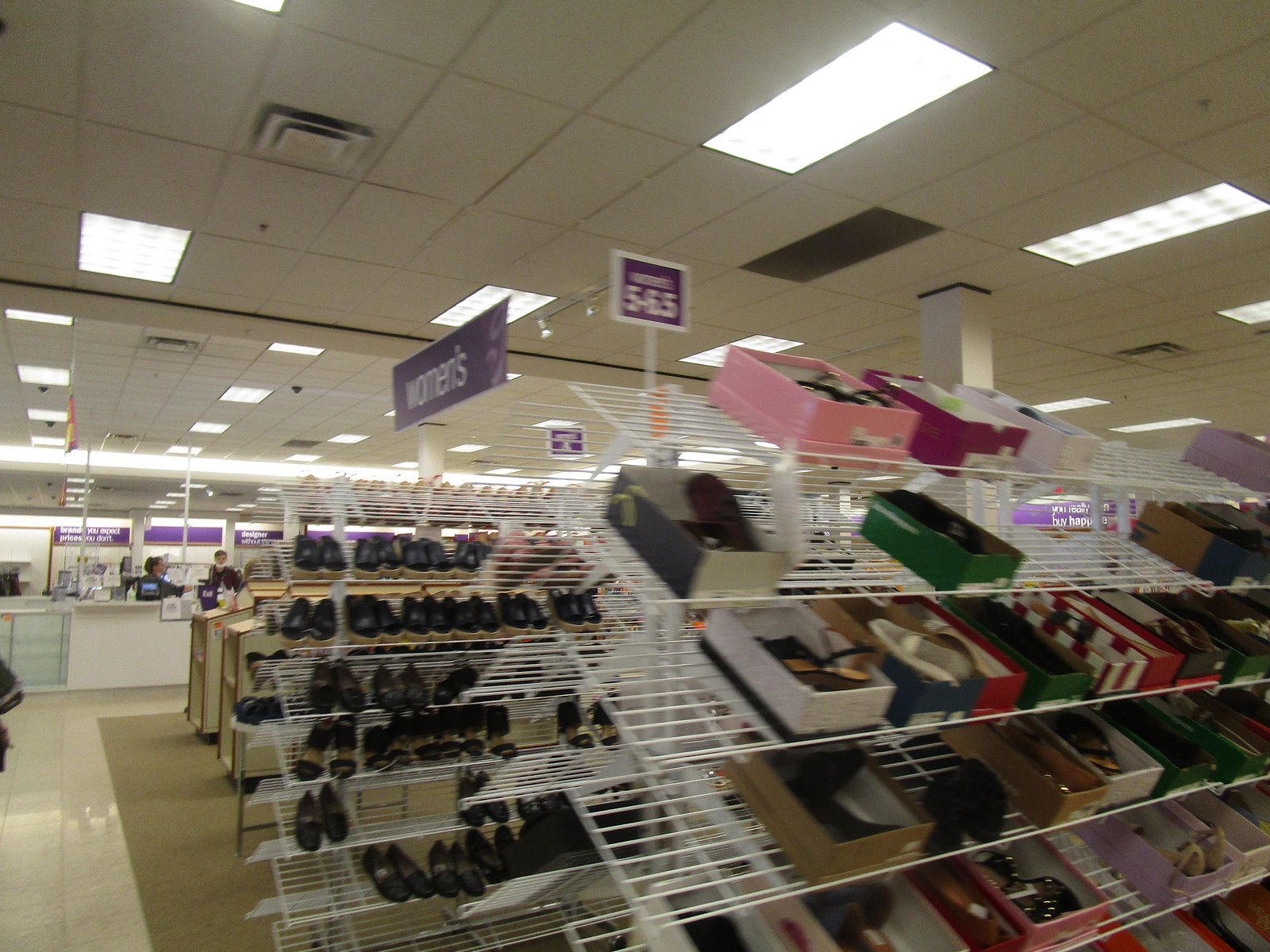Inside the women's shoe department of a bustling department store, rows of meticulously organized shoe racks greet shoppers. These racks feature a mix of shoes displayed neatly out of their boxes and others still nestled inside. Designed to enhance visibility, the racks are slanted, making each pair easily accessible. The entire shoe section rests on plush carpet, providing comfort for those browsing, contrasted by the linoleum flooring in the aisles between sections.

In the background, a sleek white counter, partially encased in glass, stands with at least one attendant behind it, ready to assist customers. Overhead, vibrant purple signs indicate the various shoe sizes available, specifically marked from sizes 5 to 6.5. The signs clearly designate this area as the women's shoe section, offering a straightforward and organized shopping experience. The overall atmosphere is typical of a well-maintained, mid-range department store, balancing functionality with a touch of comfort.